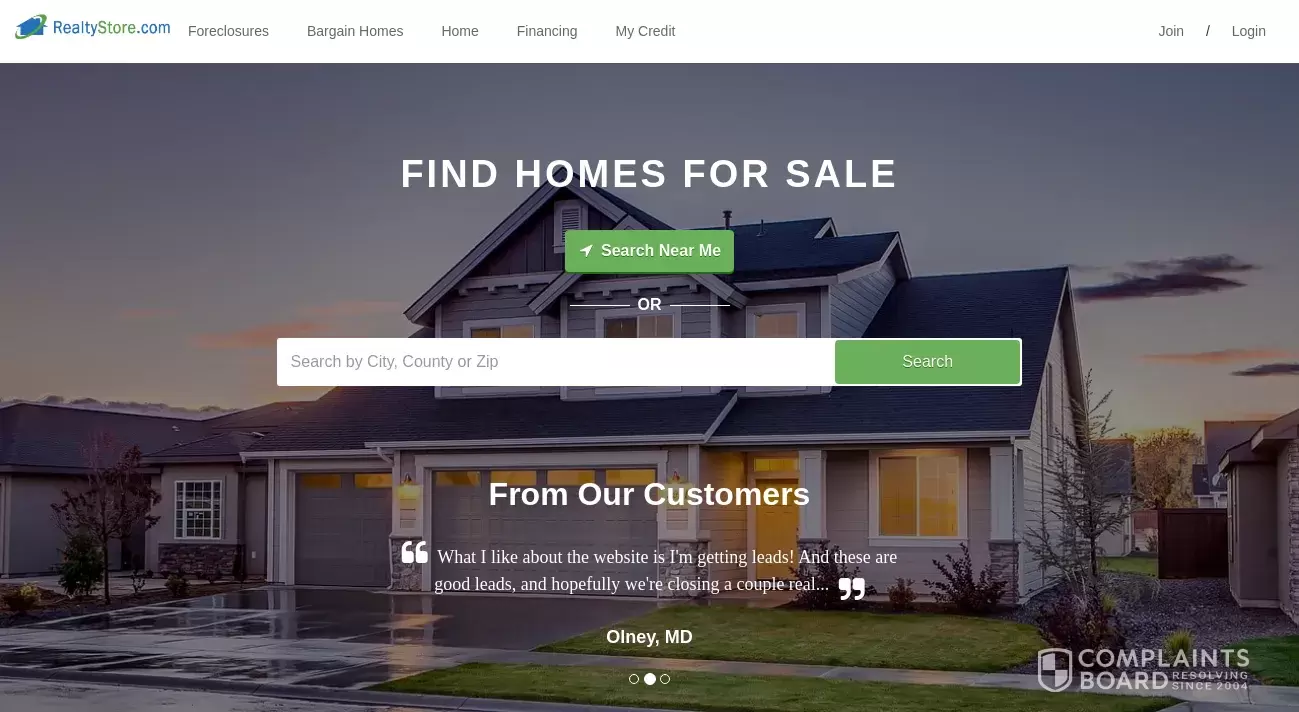This image appears to be a promotional visual for a real estate website. It is a horizontal, rectangular photo of a two-story house with a three-car garage, painted in a gray hue. The background features a serene, near-sunset sky with a few scattered clouds, creating a calming ambiance as daylight fades. At the top of the image, white text reads, "Find homes for sale." Overlaying the picture of the house, there is a green rectangle containing the words "Search near me," accompanied by a search bar prompting users to "Search by city, county or zip." Adjacent to the search bar is a clickable search button. Beneath this, user testimonials are introduced with the phrase, "From our customers." A testimonial snippet follows: "What I like about the website is I'm getting leads and these are good leads and hopefully we're closing a couple real..." The testimonial is attributed to a user from Olney, Maryland. In the bottom-right corner, a white shield symbol with the text "Complaints Board resolving since 2004" is displayed.